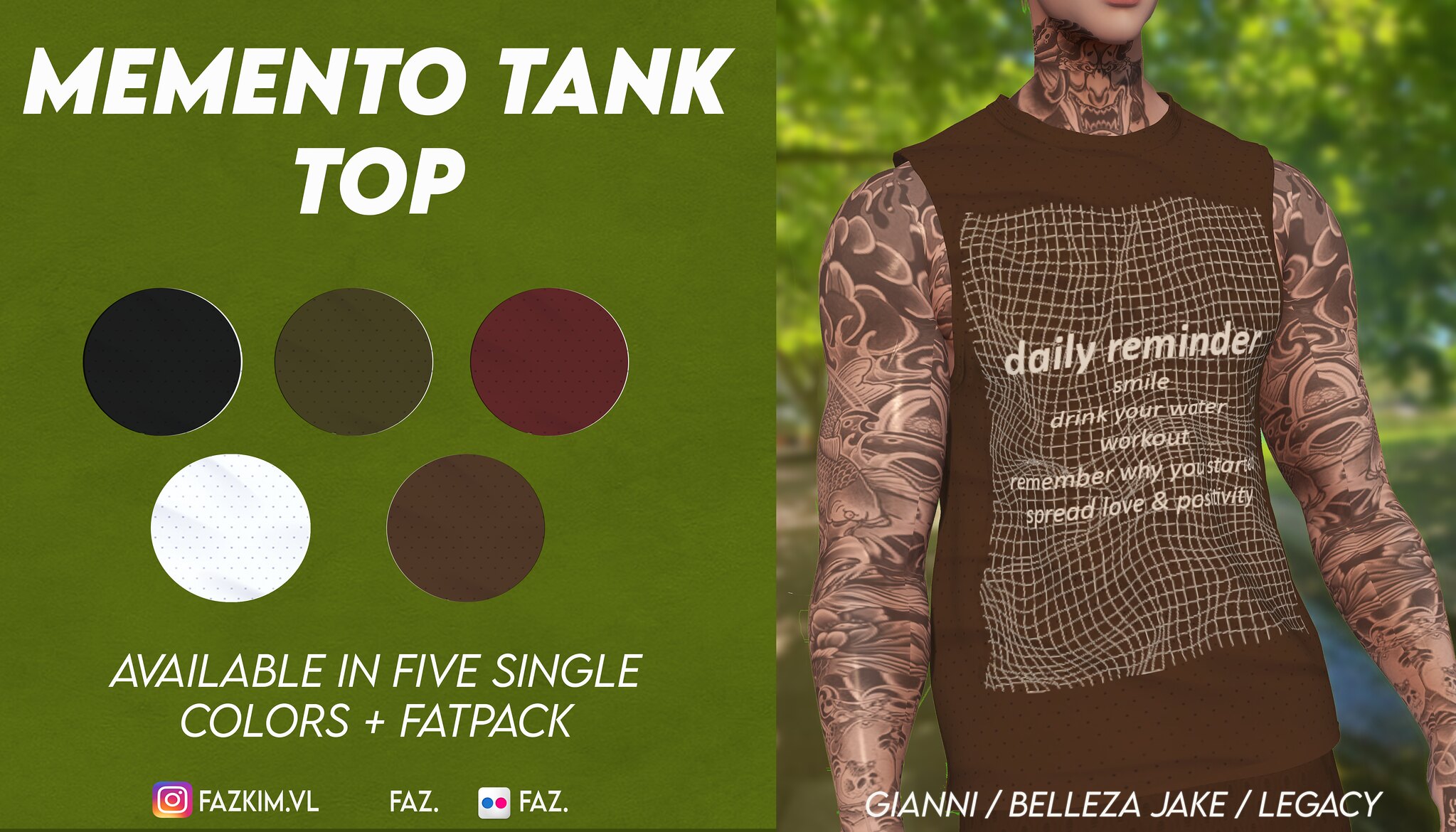This advertisement image is split into two sections. The left side features a dark green background with bold white text that reads "Memento Tank Top." Below this text, there are five circles displaying different color options: blue, green, magenta, white, and brown. The text underneath the circles states "Available in five single colors and Fat Pack." Additionally, the Instagram handle "FazKim.VL" is displayed along with the username "FazDot" beside a square logo with a blue and pink dot.

On the right side of the image, there is a person modeling a sleeveless black tank top. This tank top features a wrinkly grid design with white lines, resembling folded graph paper. Superimposed on this design, in white text, are motivational reminders: "Daily reminder: Smile, drink your water, workout, remember why you started, spread love and positivity." The model's head is cropped out above the chin, revealing heavily tattooed arms and neck. Beneath the text, the names "Gianna, Bielsa, Jake, Legacy" are listed.